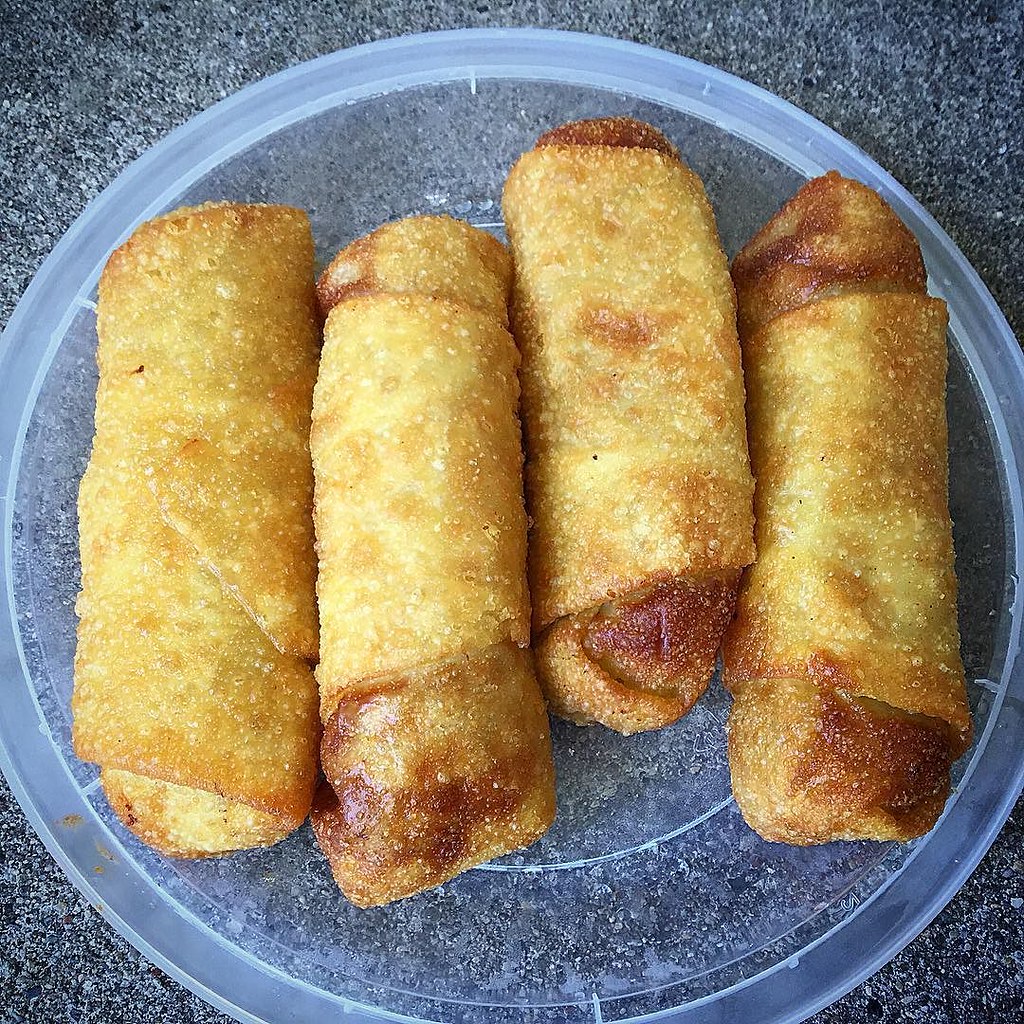The photograph features a clear, off-white plastic plate, or possibly the lid of a takeout container, prominently placed on a light gray granite countertop speckled with darker gray, resembling cement. On the plate are four freshly fried egg rolls, golden brown in color with the three on the right showing darker brown edges. The egg rolls are arranged lengthwise from bottom to top, staggered in such a way that the two on the left are nearly aligned, the second slightly lower, the third pushed higher towards the top, creating a noticeable gap, and the fourth aligned with the others. The clear lid allows the speckled countertop to be visible underneath and around the edges of the plate, adding texture to the background. The image appears to be well-composed, centered, and possibly taken in a kitchen or lunchroom setting.